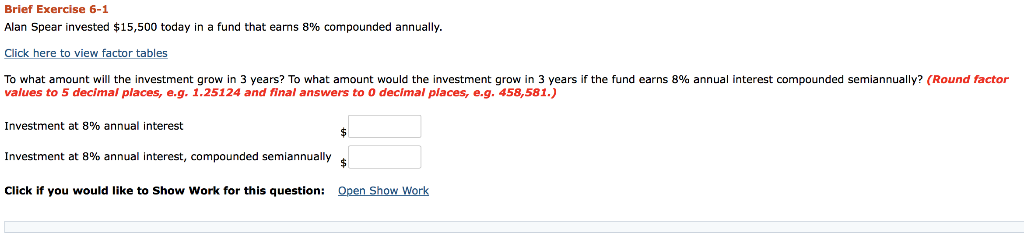The image features a white background with text presented in three different colors: red, black, and blue. At the bottom of the image, the text "Brief Exercise 6.1" is written in red. Below this, in black text, it reads: "Alan Spear invested $15,500 today in a fund that earns 8% compounded annually." This is followed by blue text that states: "Click here to view vector labels."

Further down, the text continues in black: "To what amount will the investment grow in three years? To what amount would the investment grow in three years if the fund earns 8% annual interest, compounded semi-annually?" Beneath this is another black line of text: "Round factor values to five decimal places, e.g., 1.25124, and final answer to zero decimal places, e.g., 45,581."

Following these instructions, there are additional lines in black text that provide spaces for answers:
- "Investment at 8% annual interest" with a space for the answer to be filled in on the center-right side.
- "Investment at 8% compounded semi-annually" with another space for the answer.

At the very bottom, there is a blue text prompt that instructs: "Click if you would like to show work for this question. 'Open Show Work'."